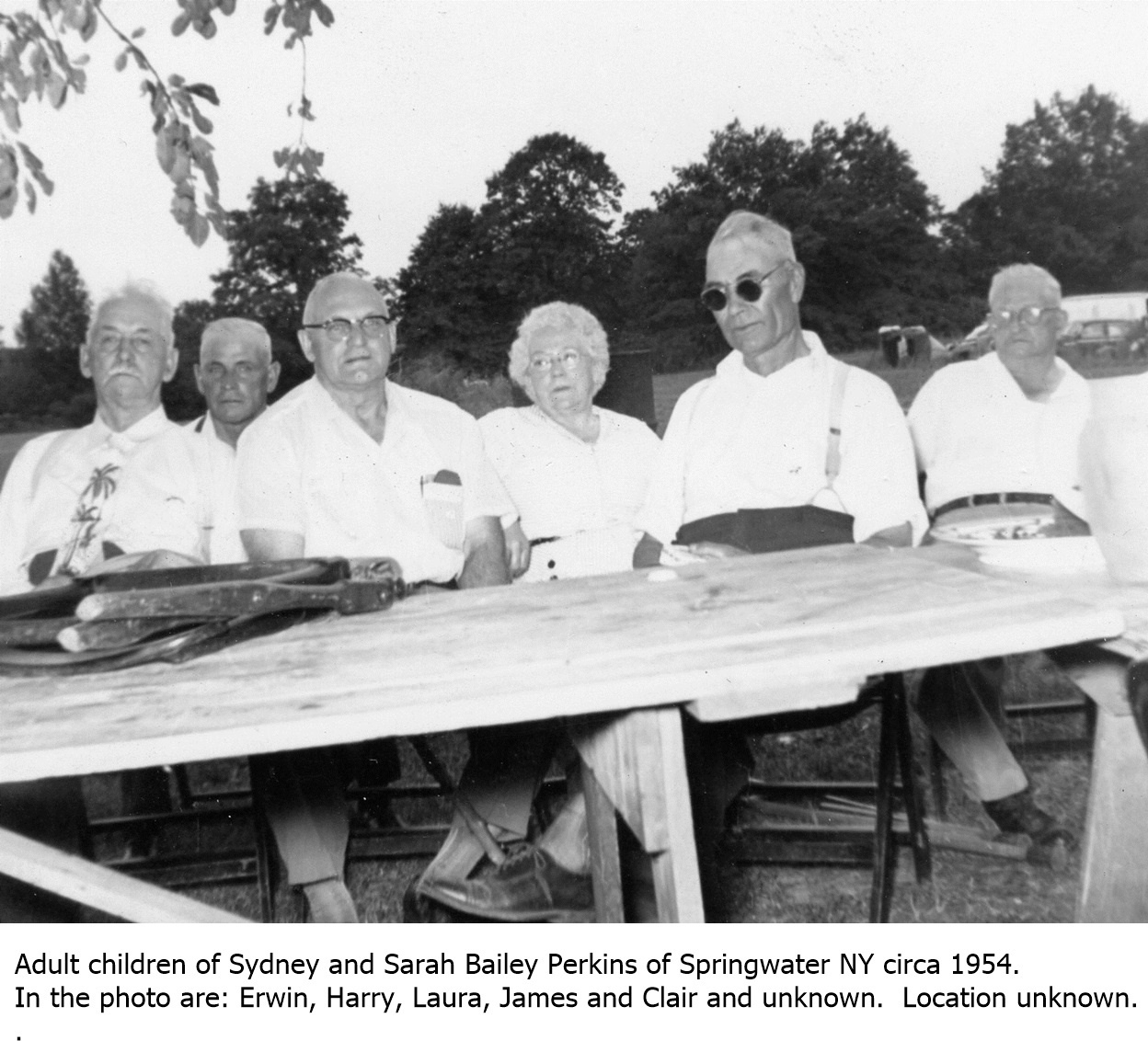In this detailed black-and-white photograph taken circa 1954, a group of older adults, identified as the children of Sydney and Sarah Bailey Perkins of Springwater, New York, is depicted sitting at a wooden picnic table beneath a tree. Labeled beneath the image as "Adult Children of Sydney and Sarah Bailey Perkins of Springwater, N.Y. circa 1954. In the photo are Irwin, Harry, Laura, James, and Claire, and Unknown.” The six individuals, five men and one woman, are dressed in white shirts. The woman, Laura, seated centrally, has short white hair and glasses. Among the men, one is distinguished by wearing sunglasses and suspenders. The wooden picnic table, showing its slatted top and a folding wooden chair positioned at the top left of the table, features some indistinct items. Tree branches hang over the left side, providing shade, while a house and a car are vaguely visible in the background behind a line of trees. The photograph captures a familial moment outdoors, set in an unspecified location, characterized by its casual, yet timeless feel.